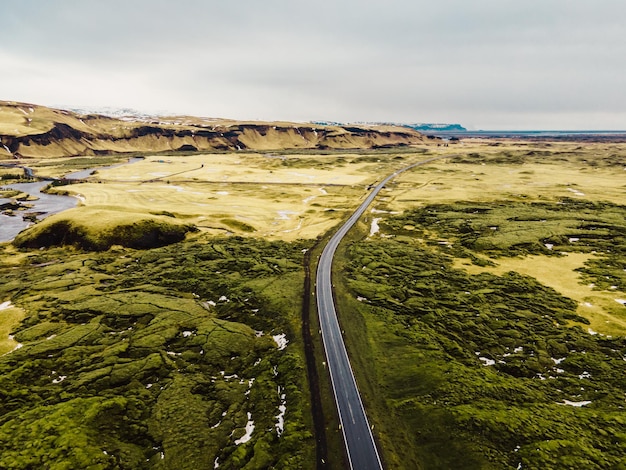The image showcases a relatively high-altitude, aerial view of a lone highway stretching into the distance through lush marshlands. Predominantly green in the foreground, the scene transitions into lighter yellows and browns towards the horizon. To the left, a larger waterway or river curves gently along the edge of the frame, merging with the interspersed wetlands. Darker patches of algae-green waters dot the landscape, hinting at the marshy terrain interspersed with sparse vegetation. Off in the distance to the right, a series of low, sloping hills in a striking yellowish hue come into view, contrasting with the overall green expanse. The horizon features a faint dark line, possibly indicating distant land or water. Above and beyond the road lies a larger body of water, so vast and faint it could be mistaken for a backdrop against the open expanse. The scene is serene and open, with subtle impressions of fertile land bordered by the continuous road that seamlessly bisects this picturesque, wetland valley.